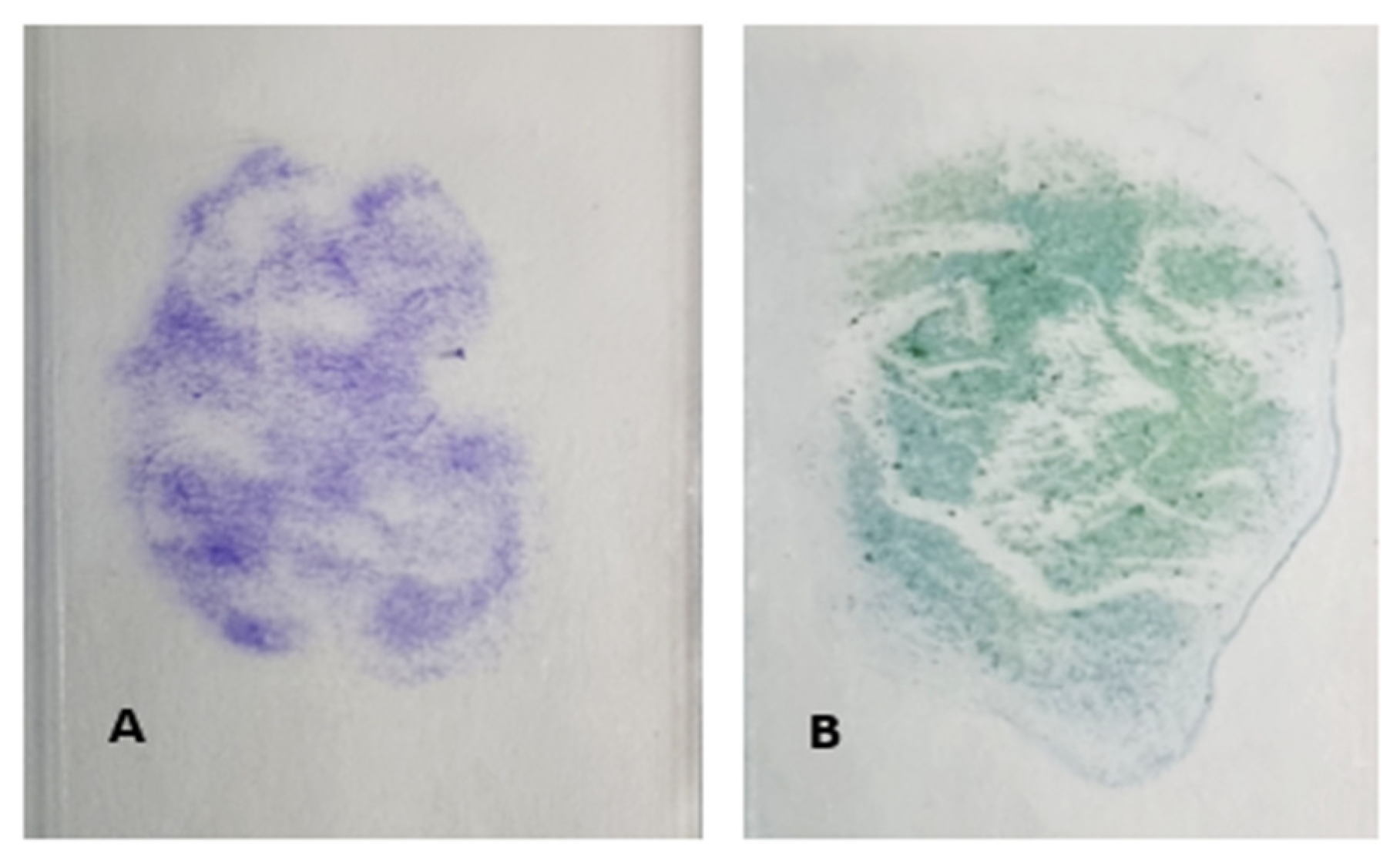The image consists of two pictures side by side on white backgrounds, each labeled in the bottom left-hand corner; the left image is marked as 'A' and the right image as 'B.' Both images exhibit a faint, almost chalk-like or spray paint appearance, characterized by distinct, slightly amorphous smudges. The picture labeled 'A' features a purple, lightly sprayed figure with an indistinct, circular pattern. It appears very faint, almost blending into the white background. In contrast, the picture labeled 'B' is a darker tealish-green color, larger than 'A,' and slightly more pronounced against the white backdrop.

Upon closer inspection, 'B' reveals a more definitive shape, which some observers might discern as the white silhouette negative of a face. This faint outline might suggest the head of a human or possibly a cat, with eyes, a nose, and a mouth potentially becoming more apparent upon prolonged viewing. Despite the similarities in their sprayed appearance, the images do not share an exact shape or pattern but are united by their ethereal, smudge-like forms.